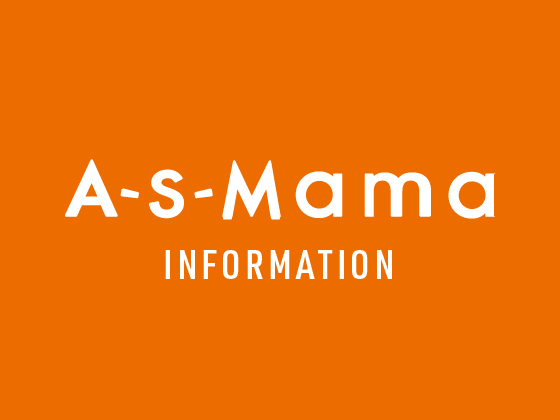The image features a logo set against a vivid and robust orange background, reminiscent of a burnt or timu orange. The logo prominently displays the text "A-S-MAMA" in white, with a mix of upper and lowercase letters; specifically, 'A-S-M' are uppercase, while 'a-m-a' are lowercase. The dashes flanking the 'S' are angled, with the left dash inclining downwards and the right dash inclining upwards. Directly beneath this, the word "INFORMATION" appears in bold, uppercase, block letters, also in white, but in a slightly smaller and different font than the main "A-S-MAMA" text. The overall design is centered and the white text contrasts sharply with the dark, vibrant orange backdrop.